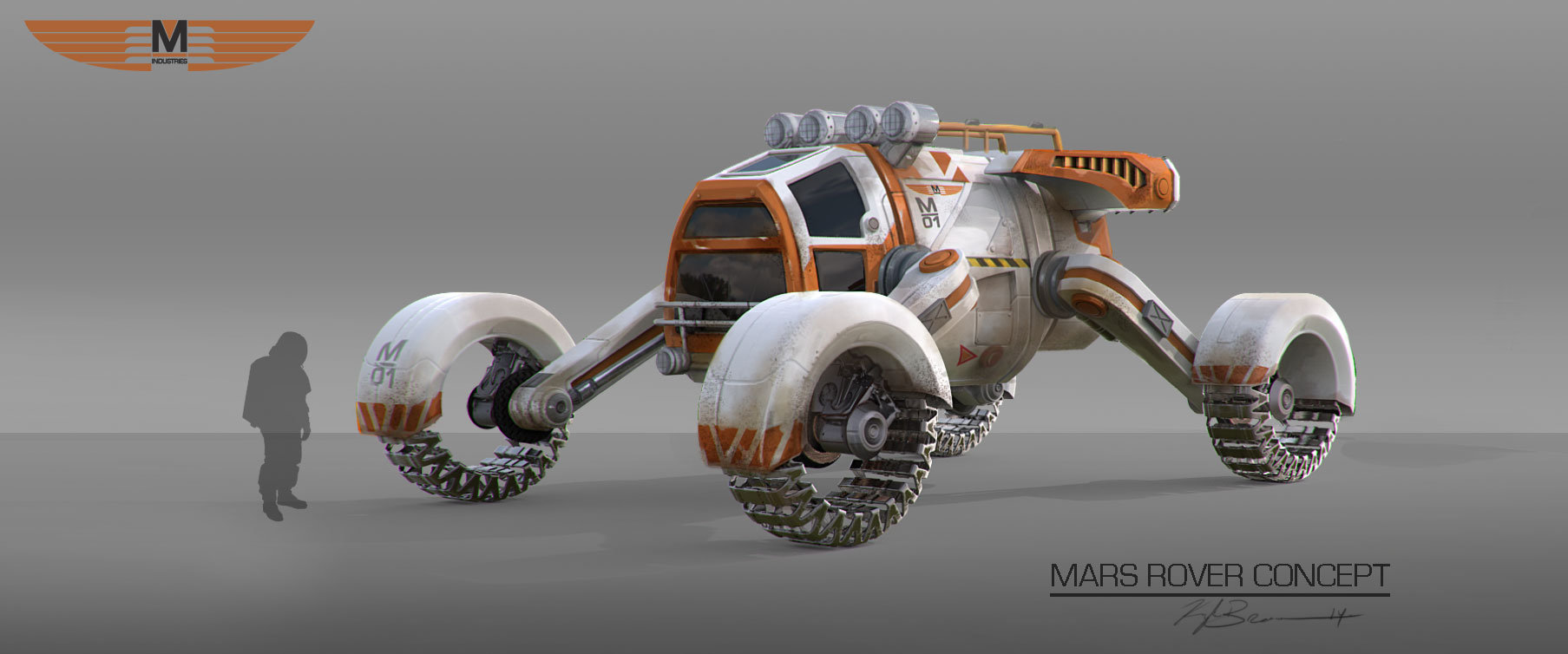The photograph showcases a Mars Rover Concept, a strikingly large vehicle with a futuristic design. The imposing machine features four circular, track-like wheels, each covered by white fenders with brown accents at the ends. On the vehicle's front passenger side, a prominent grey letter "M" sits above the number "01." The cockpit of the rover is painted in orange and white and is equipped with four round silver lights on top, complemented by metal safety bars on the hood. A silhouette of a person stands near the right front tire, emphasizing the vehicle's immense size in comparison. The image is labeled at the bottom right with the text "Mars Rover Concept" in cursive black lettering, underlined with a signature, likely of the artist. The upper left corner displays an emblem featuring a capital "M" with orange lines extending outward, reminiscent of stylized wings.